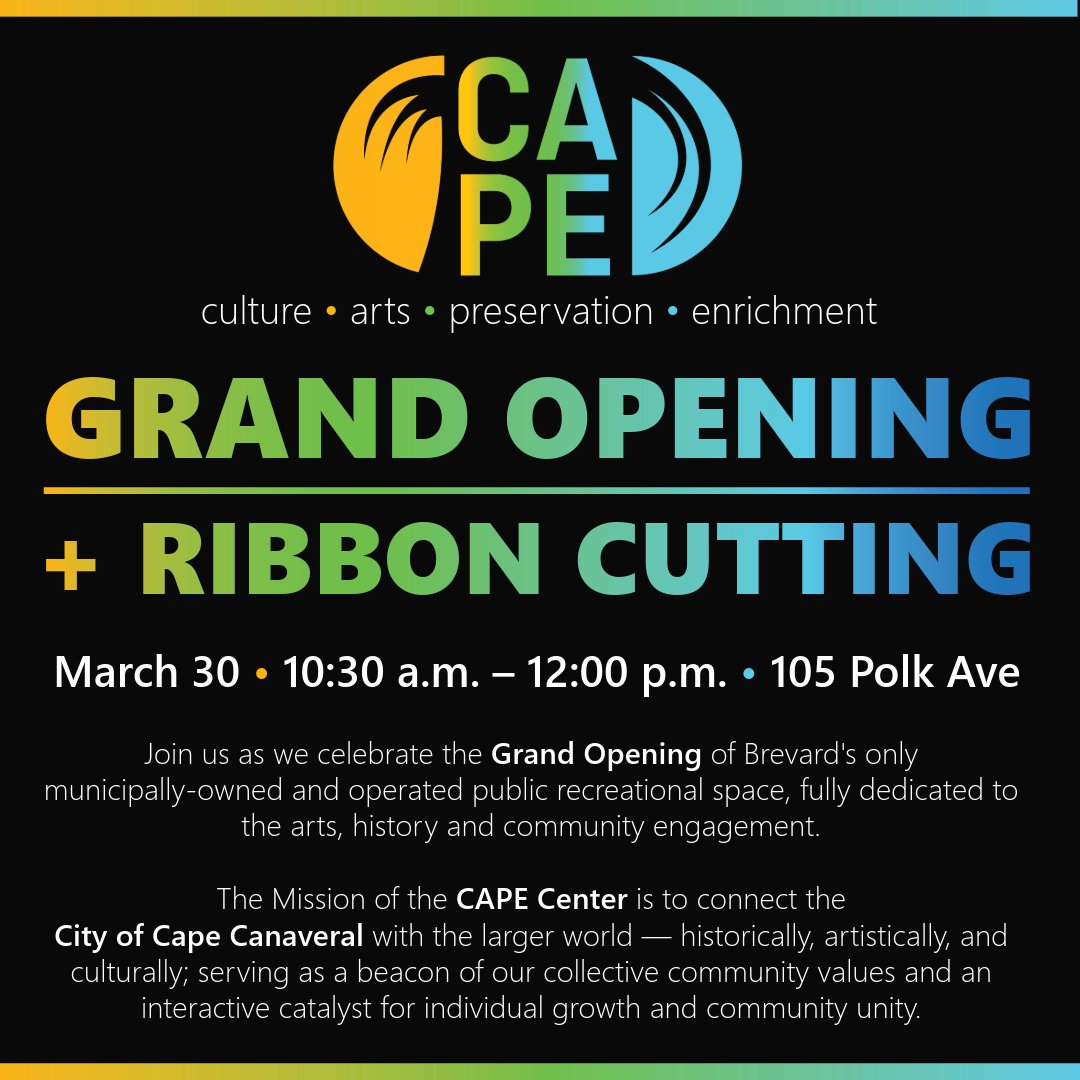This square-shaped image features a poster with a black background. Along the top and bottom edges runs a thin stripe that transitions in a color gradient from orange on the left, through yellow and green in the middle, to blue on the right. At the top, there is a logo that says "CAPE," arranged with "C.A." on top and "P.E." underneath, with a semi-circle on the left and another on the right, featuring black swirls. 

The central text on the poster follows the same gradient color scheme, starting with yellow on the left, moving to green, light blue, and ending with dark blue on the right. This text announces "Grand Opening + Ribbon Cutting." Below it, in white font, it reads "Culture Arts Preservation Enrichment," with each word separated by a small colored dot. Further down, the information continues in white: "March 30, 10:30 AM to 12 PM, 105 Polk Avenue."

The poster invites viewers to join the celebration of the grand opening of Beverage's only municipally owned and operated public recreational space dedicated entirely to the arts, history, and community engagement. The mission of the CAPE Center is to connect Cape Canaveral to the broader world historically, artistically, and culturally, serving as a beacon of community values and fostering individual growth and community unity.